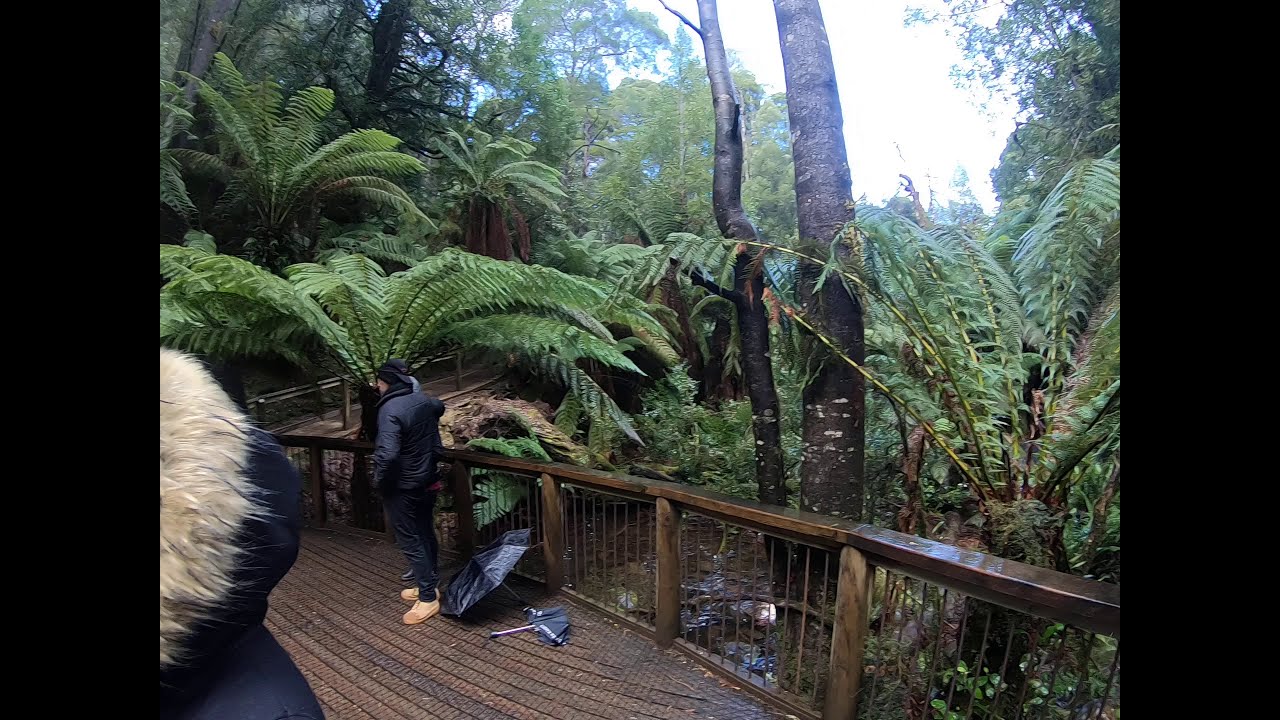The image captures a rainy scene within what appears to be a botanical garden or dense forest, featuring an elevated wooden walkway. The walkway, which has a metal bottom dirty with a mix of brown and black, is bordered on the right by a wooden railing supported by posts, with thin metal bars in between. The wood of the barrier looks soaked from the rain. Vegetation is abundant and tropical, with ferns and long-branched plants having finger-like leaves. Two people are present on the walkway, both facing away from the camera. One person stands in the center dressed in a black jacket and pants with yellow shoes, next to an open umbrella lying on the ground. The other person, partly outside the frame on the far left, is clad in a dark coat with a fur-lined hood or collar and tan boots. Both individuals and the surrounding plant life, including two slightly curved trees at varying thicknesses, appear wet from the rain. In the background, sunlight attempts to penetrate the dense canopy, creating a diffused white glow.